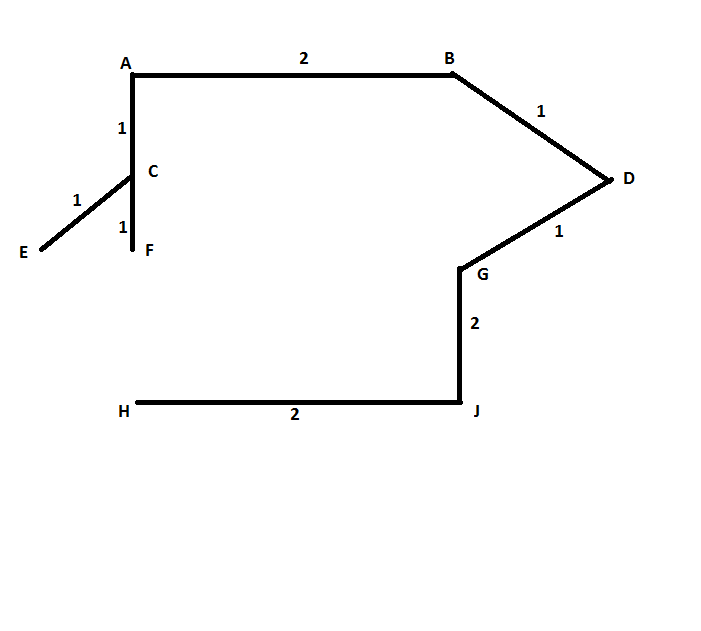The image depicts a simple black line drawing with capital letters and numbers strategically placed along various lines. Here's a detailed breakdown from bottom to top and left to right:

1. **Bottom Line**: A straight horizontal line spans the width of the image. Starting from the left:
   - The letter **H** is situated at the very beginning.
   - Approximately halfway along this bottom line is the number **2**.
   - At the extreme right end of this bottom line is the letter **J**.

2. **Vertical Ascent**:
   - From the end of the bottom line (near the letter J), a vertical line extends straight up.
   - At the midpoint of this vertical line is another number **2**.

3. **Diagonal Line Upwards**:
   - From the top of the vertical line, a diagonal line extends slightly upward to the left.
   - At the starting corner of this diagonal line (connected to the vertical line) is the letter **G**.
   - Midway along this diagonal line is the number **1**.
   - At the end point of this diagonal line is the letter **D**.

4. **Top Horizontal Line**:
   - From the end of the diagonal line (near the letter D), another horizontal line extends to the left.
   - Along this top line, roughly midway is the number **1**.
   - At the top left corner (where this horizontal line starts), the letter **B** is placed.
   - The middle of this line contains the number **2**.
   - At the far left end of this top horizontal line is the letter **A**.

5. **Descending Vertical Line**:
   - From the letter A, a vertical line drops straight down.
   - This line aligns vertically with the starting point at the bottom (where H is located) but does not reach the bottom, stopping halfway.
   - The left-hand side of this descending line features the number **1**.
   - Slightly below halfway down this vertical line, the letter **C** is on the right-hand side.

6. **Lower Diagonal Line**:
   - From this same vertical line near C, another diagonal line proceeds downward to the left.
   - This diagonal line includes the number **1**.
   - At the end point of this lower diagonal line is the letter **E**.

7. **Final Vertical Segment**:
   - Returning to the main vertical line (from the letter A), along this line near its lower segment, there is another number **1**.
   - Finally, at the bottom of this vertical line is the letter **F**.

This detailed structural description captures the intricate layout of letters and numbers, despite the unclear purpose of the drawing.